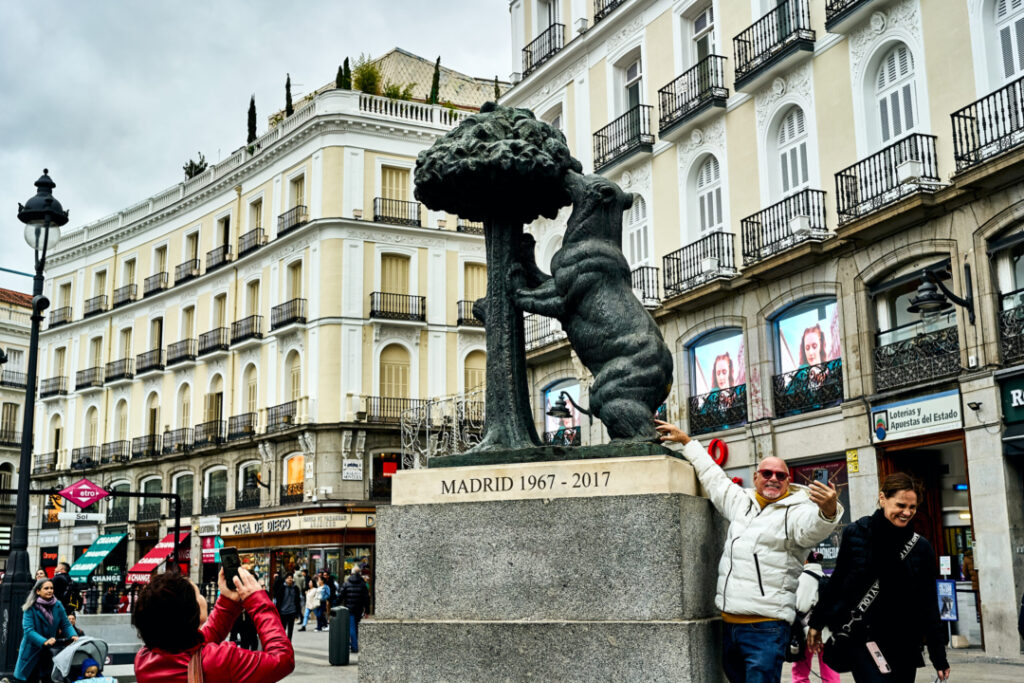The landscape photograph captures a lively scene in a bustling Madrid square, dominated by the striking statue of a bear standing upright, reaching into the dark green foliage of a tree, which symbolizes Madrid and commemorates the years 1967 to 2017. The bronze sculpture rests on a concrete base, drawing the attention of several onlookers. 

In the foreground, a bald man in a white puffy coat and red sunglasses poses for a selfie, his right arm extended towards the bear while the left hand holds his phone. Next to him, a woman in a blue coat with pulled-back blonde hair and a purple scarf pushes a baby carriage, where a baby wearing a blue hat peeks out. Nearby, another woman with light skin and brown hair dressed in a red coat holds up her phone to capture the scene.

The background features characteristic light yellow and white apartment buildings, about four stories high, each adorned with black balconies and rounded archways. Between the buildings, storefronts line the street level, adding to the urban ambiance. The sky above is overcast, casting a muted light over the entire scene, and on the top left corner of the image, a black streetlight with a glass bulb stands out. The public square is a hive of activity with people walking around, engaging with the sculpture, and savoring the lively atmosphere of the city.